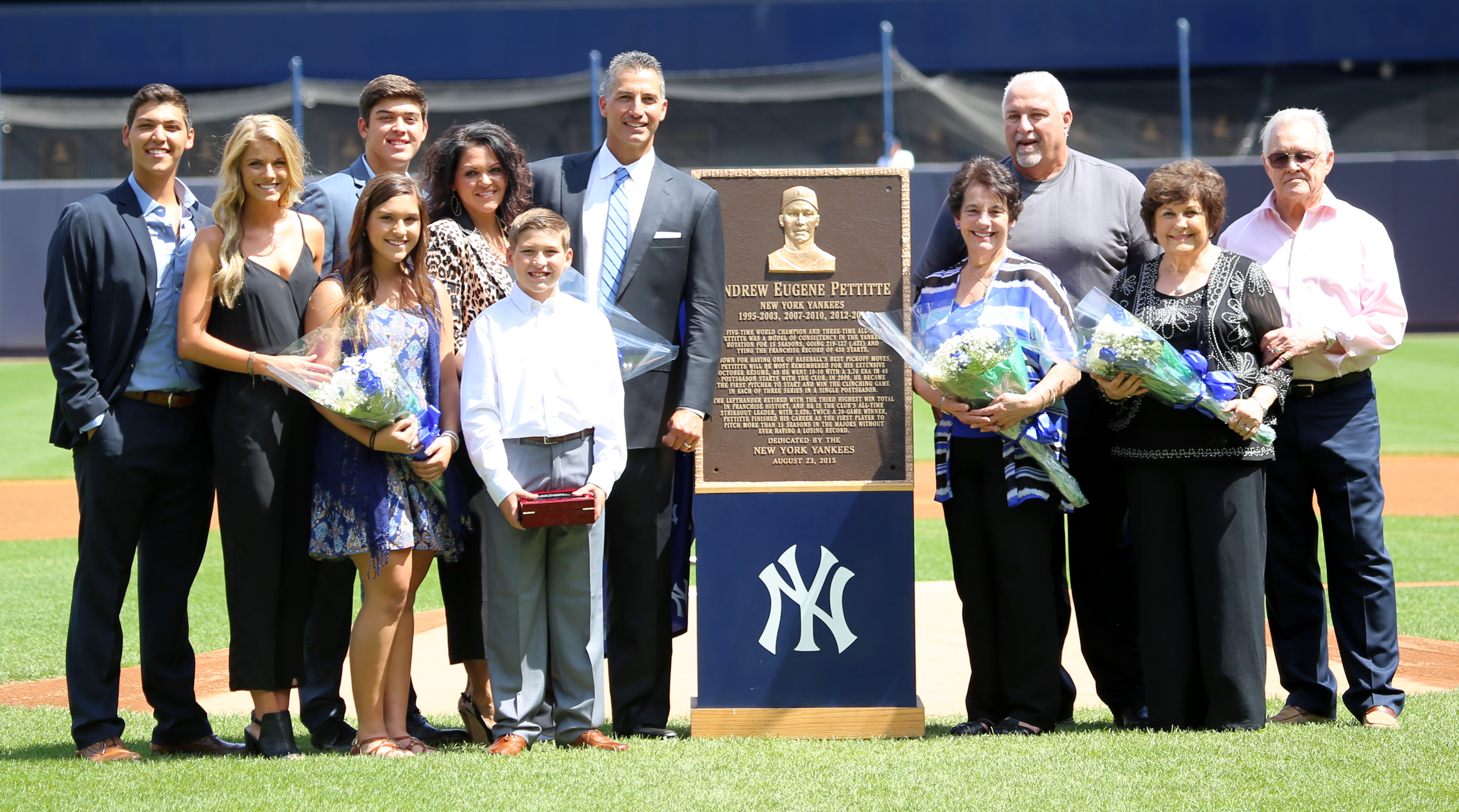The image shows a vibrant scene set on a baseball field under the midday sun. The ground is covered in a mix of flat grassy areas and scattered dirt mounds, typical of a baseball field. In the background, you can see the home run wall and protective nets, with stands for spectators further back. Dominating the center of the image is a tall, person-sized memorial plaque with a wooden base. The plaque features a New York Yankees logo in white on a blue background, and above it in gold lettering, it reads "Andrew Eugene Pettitte." The plaque includes additional text and dates, though they are not clearly legible, and a golden portrait of Pettitte is prominently displayed above.

Surrounding the monument, a group of people, likely family members and possibly stadium staff, are gathered for what appears to be a dedication ceremony. To the left of the plaque, older individuals in suits and holding bouquets of flowers stand solemnly, while younger children, possibly holding an urn, stand nearby. Off to the right, more people, some holding flowers as well, are present. The entire scene suggests a moment of commemoration and remembrance, with a diverse group of attendees consisting of relatives and ballpark personnel. The setting and solemn arrangement of individuals indicate a significant dedication event honoring Pettitte.